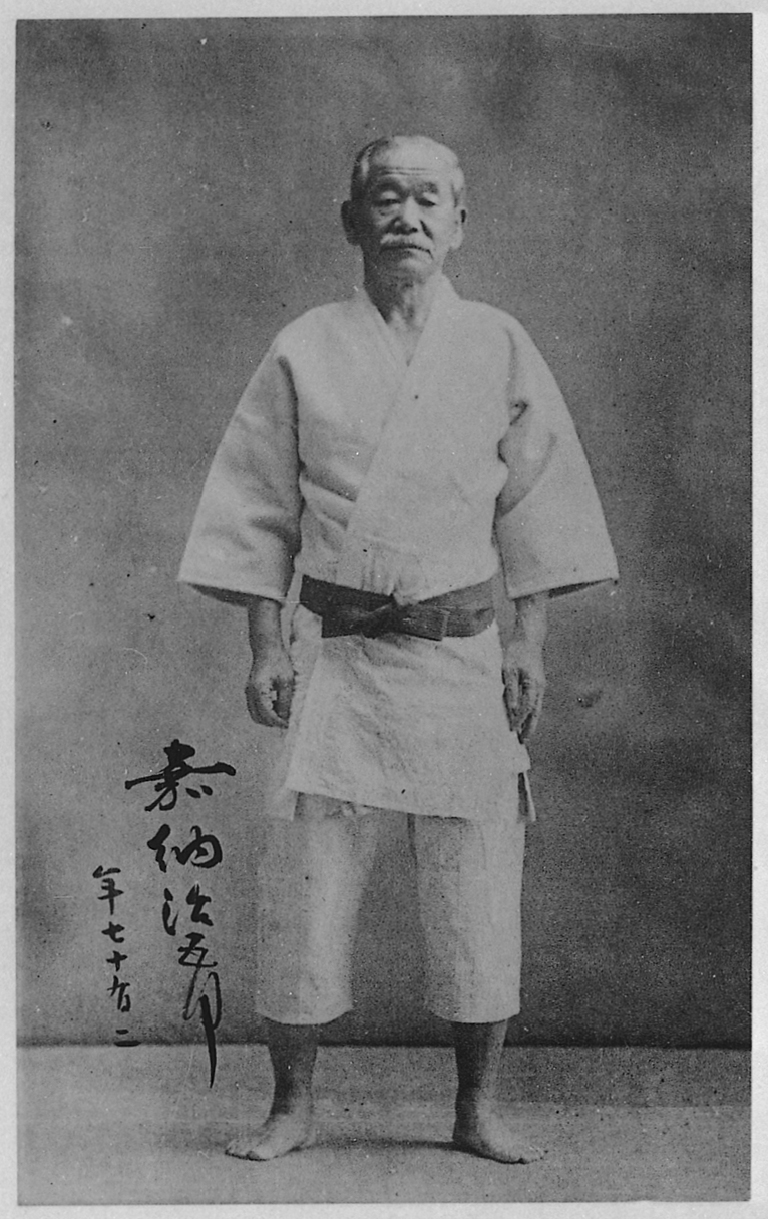This black-and-white photograph captures an elderly martial arts master, possibly specializing in Kung Fu or a similar discipline, standing confidently in the center of the frame. The man, who is partially bald with a white mustache, appears relaxed with his feet slightly apart and his hands resting by his sides. He is dressed in a traditional white Kung Fu outfit that reaches his calves, secured by a darker belt tied around his waist. The background is plain, making the master the focal point of the image, and the photograph seems to be quite old, indicated by its appearance and the gray border framing it. To the left of the master, there is Asian text, most likely Japanese or Chinese, which might include his name or title. The simplicity of the setting—void of any distracting elements—and the focus on the martial artist suggest a moment of calm and dignified stature, emphasizing his long-standing expertise in martial arts.